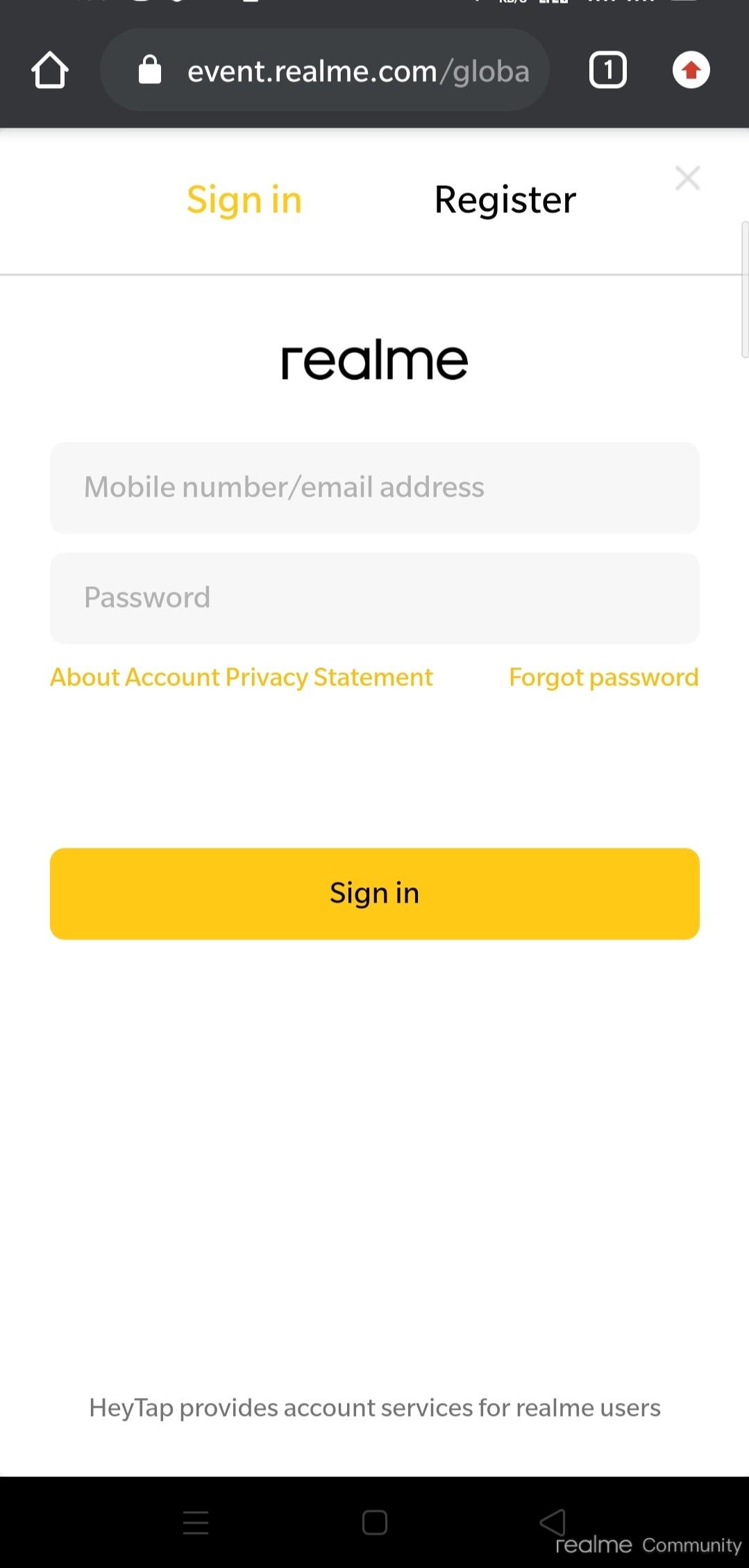The image displays a smartphone screen in portrait mode, featuring a login page for Realme's event website. At the top left of the screen, there is an icon depicting a small white house. On the top right, an address bar with a white padlock icon indicates the URL: event.realme.com, though the "global" part of the URL is partially cut off. There is one active tab indicated by the number "1" in a white box. Next to it is a white circular button with a red arrow pointing upwards.

Below this section, a prominent white area contains two main action buttons: a yellow "Sign In" button and a black "Register" button. An "X" icon is located in the upper right corner of this section. Directly underneath, the brand name "Realme" appears in black text. The login form comprises two gray-text placeholders within text boxes—the first for a "Mobile Number/Email Address" and the second for a "Password."

Further down, in yellow text, links to the "Account Privacy Statement" are present, with a "Forgot Password" link in black text to the right. Beneath this, a large yellow button with "Sign In" written in black provides a call to action. Finally, at the bottom of the screen, gray text informs users that "Haytap provides account services for Realme users." In the bottom right corner, "Realme Community" is displayed in a black section.

This detailed description captures all elements of the login interface displayed on the phone screen, ensuring clarity and comprehensiveness.